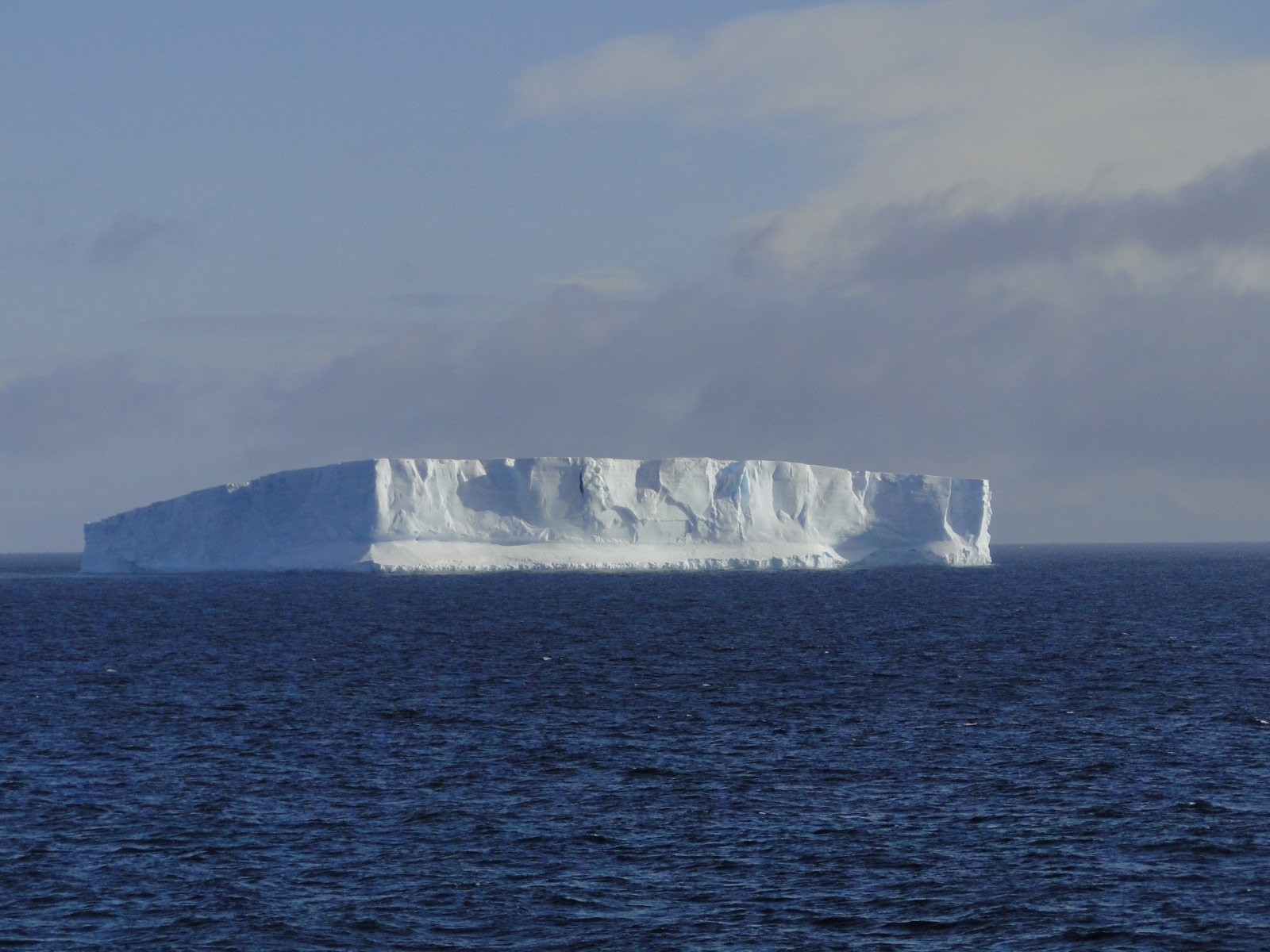In the image, a large, rectangular iceberg with jagged edges floats in the dark blue open sea. The photograph, which is nearly square, is split almost evenly between the sky and the water. The iceberg's flat top and relatively low height emphasize its width. The sun illuminates the front face of the iceberg, which also features a small black speck. Surrounding the iceberg, the sky is a gradient of blue, with a mix of pale, wispy clouds and darker gray clouds near the horizon, rising to whiter shades higher up. The water shows slight unevenness but lacks significant waves, and no land is visible in the background, reinforcing the isolation of the scene. The overall atmosphere is serene yet dramatic, with the contrasting colors of the sky, sea, and iceberg adding to the visual impact.